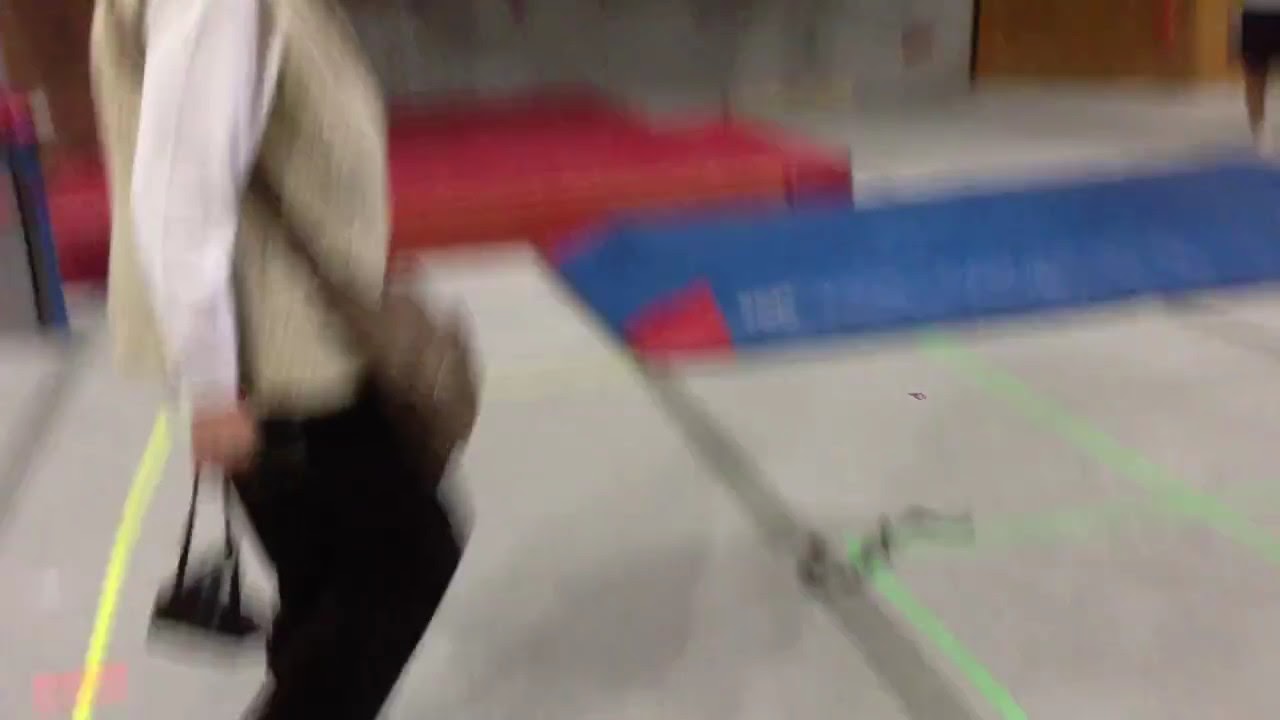The image is a blurry photograph taken with a low-quality camera. It depicts the side view of a person walking towards the right, though their head is cropped out, making it impossible to determine their gender. The person is dressed in a white long-sleeved collared shirt layered with a tan vest, along with black pants. They are carrying a brown shoulder bag. The ground beneath them appears to be made of cement slabs featuring yellow and green lines. In the background, there is a raised platform that is bright blue with red at the corner, and another red platform on top of the blue one.